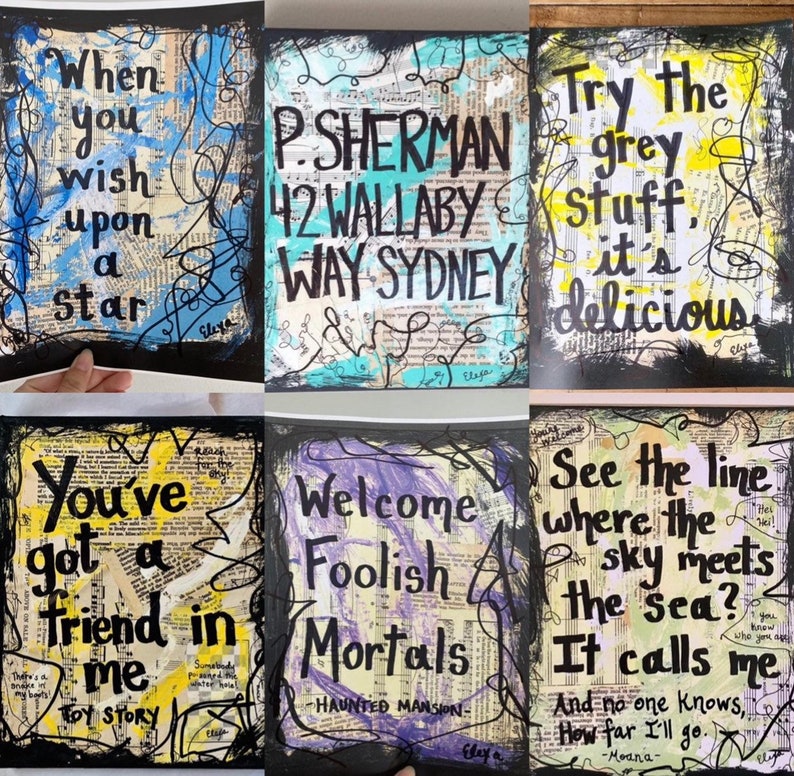The image features six distinct pieces of paper mache art styled with newspaper prints and paint, organized in two rows of three. Each piece contains a familiar phrase from Disney or Pixar movies. The top left piece, held by a hand, has a dark background with white newspaper print, blue squiggly lines, and a central phrase, "When you wish upon a star." Below it, in small letters, appears the name "Eliza." Next, a turquoise piece displays the iconic address "P. Sherman, 42 Wallaby Way, Sydney," with black squiggly lines and smears of turquoise paint. The center top piece includes yellow streaks and the phrase, "Try the gray stuff. It's delicious," with "delicious" in script and a black border. 

On the bottom left, another yellow piece with black squiggles states, "You've got a friend in me," while referencing "Toy Story" and featuring some barely legible small lettering. The middle bottom piece has purple streaks and a mottled border with the text, "Welcome, foolish mortals," and "Haunted Mansion" underneath. The final piece on the bottom right is multicolored with light shades of green, purple, and yellow. It features the line, "See the line where the sky meets the sea. It calls me and no one knows how far I'll go," possibly signed with a name starting with "M" or possibly "H," which is hard to decipher. This array of vibrant, mixed-media art celebrates beloved Disney and Pixar quotes in a creative homemade style.